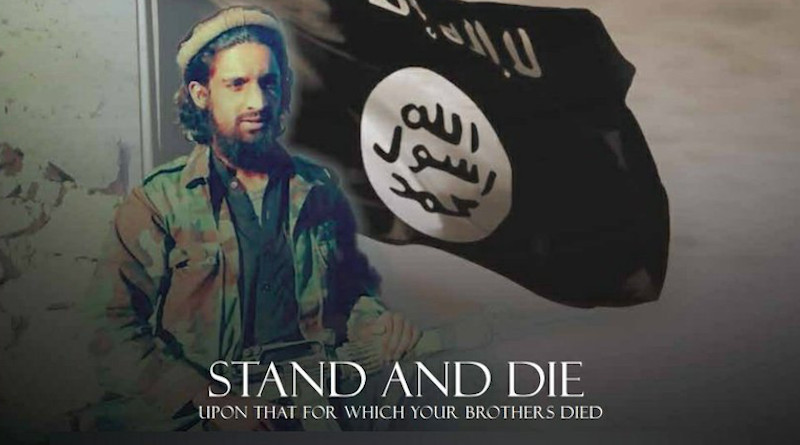The image depicts a bearded man with black hair, wearing a camouflage jacket over a black shirt, and a flat hat. He appears to be holding an assault rifle. Standing slightly right of center, he is positioned in front of a black flag featuring a yellow circle in the center, containing foreign text. The flag and the entire background are dark and stylized with blur filters, making it hard to distinguish detailed features. White text at the bottom of the image reads, "Stand and Die, upon that for which your brothers died." The overall impression suggests a militant or jihadist theme, possibly related to ISIS or a similar jihadist state.